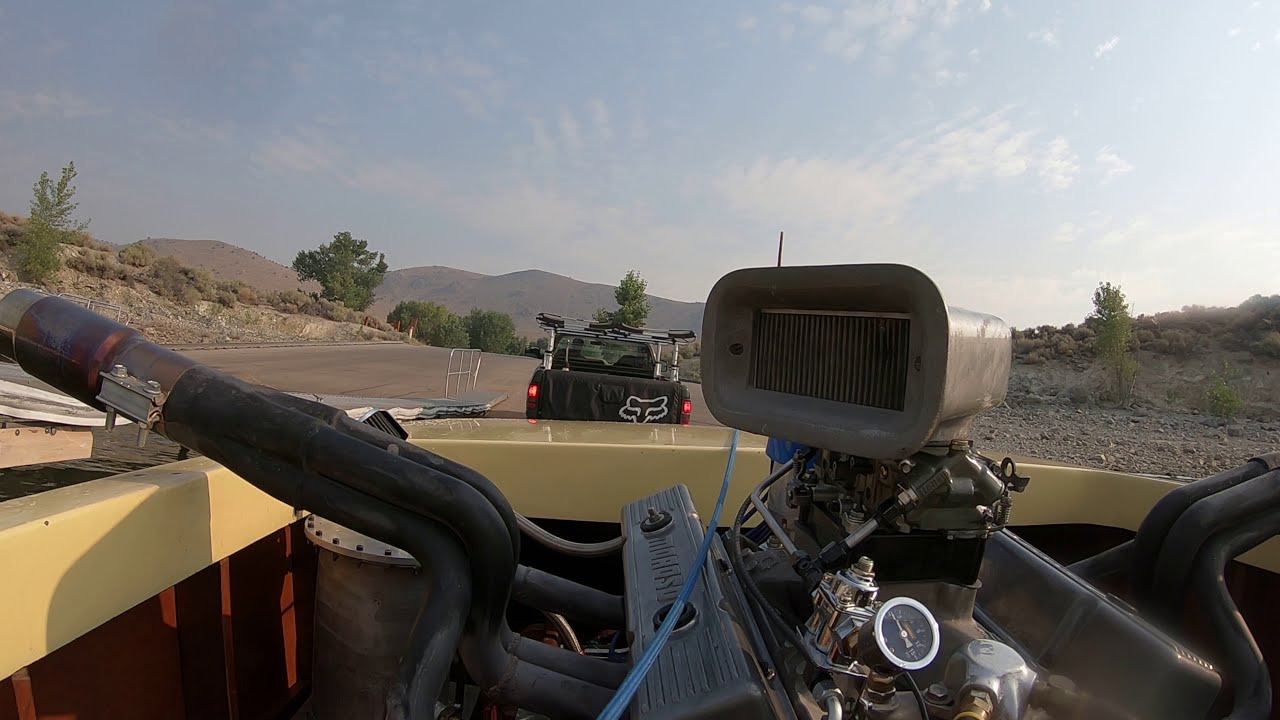The photograph showcases an outdoor scene featuring a central yellow trailer carrying a large, secured motorcycle engine with gray and silver parts, including black hoses. This trailer is being towed by a black truck with a metal frame around its bed, displaying branding from a motocross company. The road, paved and stretching into the distance, is flanked by green-leaved trees on either side and extends towards an orange and brown mountain range in the backdrop. The bright daytime setting, marked by a mostly blue sky with a few clouds, illuminates the desert-like landscape that seems reminiscent of regions like Arizona or New Mexico. Dirt trails and roads can also be seen scattered through the scenery. The scene captures a sense of movement and the rugged, open road adventure.